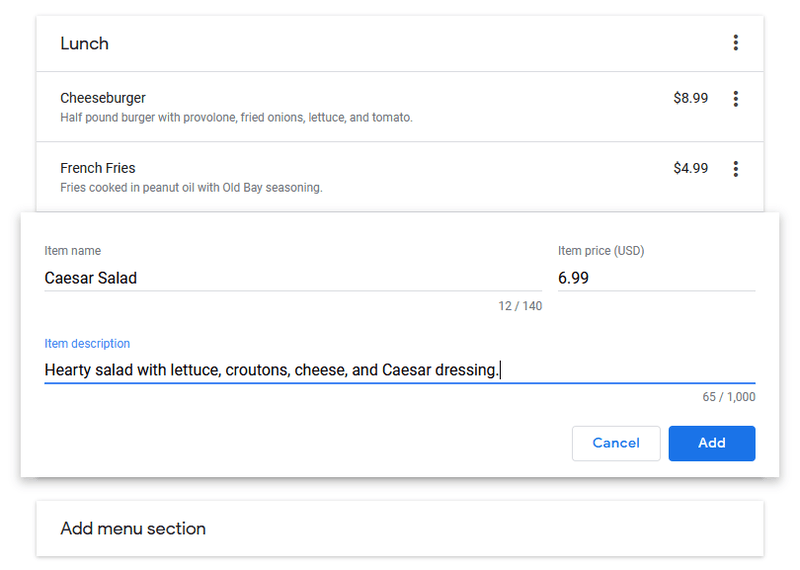The image displays a menu with a sophisticated layout. The menu is encased in a gray border and features a clean white background. Each menu item is elegantly divided by a subtle gray line. At the very top, aligned to the left, the word "Lunch" is prominently displayed in bold black text. To its right, vertically aligned, are three dots.

The first menu item listed is a "Cheeseburger." This item is described as a half-pound burger topped with provolone cheese, fried onions, lettuce, and tomato, priced at $8.99, situated on the far right. Below this, the next item is "French Fries," described as fries cooked in peanut oil and seasoned with Old Bay, priced at $4.99.

Further down, there is a larger, more detailed box that stands out from the rest of the menu. This box lists "Caesar Salad" with an item price of USD $6.99 and a notation "12 / 140." Below the item name and price, the description reads: "Hearty salad with lettuce, croutons, cheese, and Caesar dressing." At the bottom right of this larger box, there are two buttons: a "Cancel" button on the left, and an "Add" button on the right.